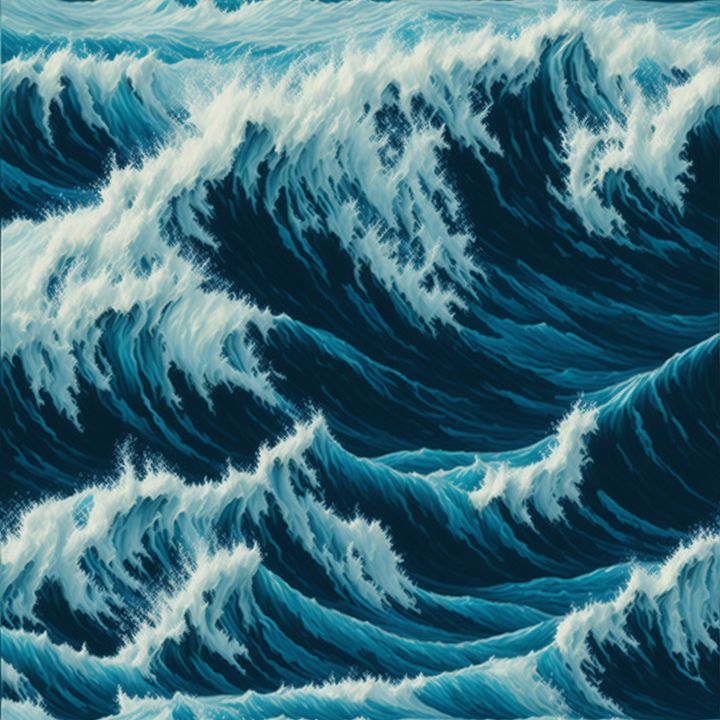This image depicts a striking painting of the ocean during a storm, showcasing large, dark blue waves that verge on black. The waves are capped with white tips and rolling swells, creating a dramatic contrast that emphasizes the turbulent sea. The artist's use of deep, thick shades of blue lends a striking realism to the scene, making the waves appear powerful and almost palpable. The foam on the waves appears white, a detail that enhances the lifelike quality of the painting. The edges of the image cut off some of the waves, adding to the impression of an expansive, tumultuous ocean. There is no text or other elements in the image, allowing the viewer to fully immerse in the intensity and beauty of the stormy seascape.